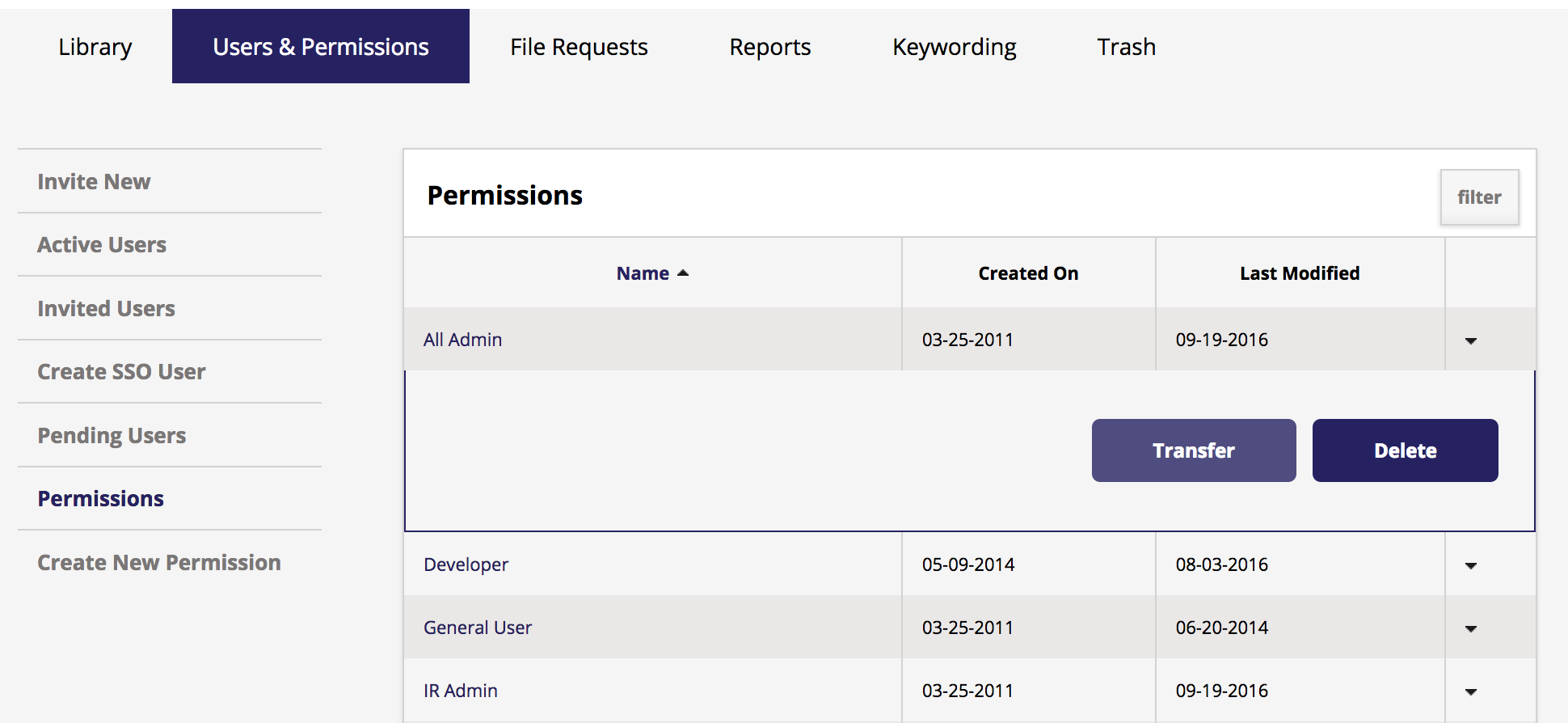The image features a comprehensive screenshot of a computer interface. It is displayed in a left-to-right horizontal format with a gray background typical of many desktop applications. 

At the top of the screen are clickable category labels in black, encased within a blue box: "Library," "Users," and "Permissions." Additional sections include "File Requests," "Reports," "Keywording," and "Trash."

On the left-hand side, there’s a vertical menu with options listed in gray text, each separated by a thin gray line. These options include "Invite New Active Users," "Invited Users," "Create SSO User," "Pending Users," "Permissions" (highlighted in purple), and "Create New Permission."

Dominating the center of the screen, the word "Permissions" appears in bold black text atop a white background. To the right, there's a clickable "Filter" button.

The main section displays a chart with columns labeled "Name," "Created On," and "Last Modified." At the end of each row, there are "Transfer" and "Delete" buttons. 

The rows in the chart are as follows:
1. "All Admin" - Created on 3-25-2011, Last Modified on 9-19-2016.
2. "Developer" - Created on 5-9-2014, Last Modified on 8-3-2016.
3. "General Users" - Created on 3-25-2011, Last Modified on 6-20-2014.
4. "IR Admin" - Created on 3-25-2011, Last Modified on 9-19-2016.

Each entry in the table is clearly separated by lines, ensuring an organized and easily navigable interface.